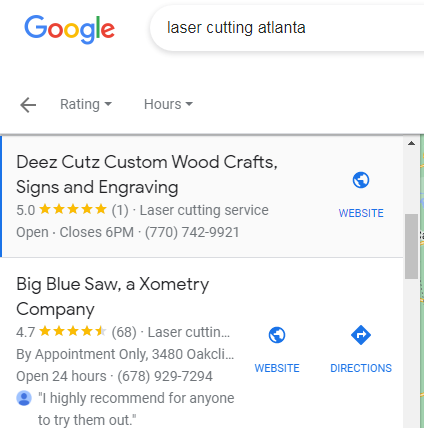A screenshot of a Google search on a mobile phone showing the search query "Laser Cutting Atlanta" is displayed. The familiar multi-colored Google logo is situated at the top left corner. Directly below the search bar heading towards the right, terms like "Rating" with a left-pointing gray arrow beside it and a drop-down menu follow. Further, "Hours" is visible, also accompanied by a drop-down menu. 

The screen lists two businesses:

1. **Deez Cuts Custom Wood Crafts, Signs, and Engraving**:
   - Rated 5.0 stars with five yellow stars and (1) review.
   - Labeled as a "Laser Cutting Service."
   - Status: Open, with closing time listed as 6 p.m.
   - Includes a phone number.
   - A button for the website is located on the far right side.

2. **Big Blue Saw, an examinee company**:
   - Rated 4.7 stars.
   - Status: Open by appointment only.
   - Provides clickable links for Website and Directions.

In summary, the visual portrays a search result page highlighting two highly-rated laser cutting services in Atlanta, featuring essential contact and operational details.